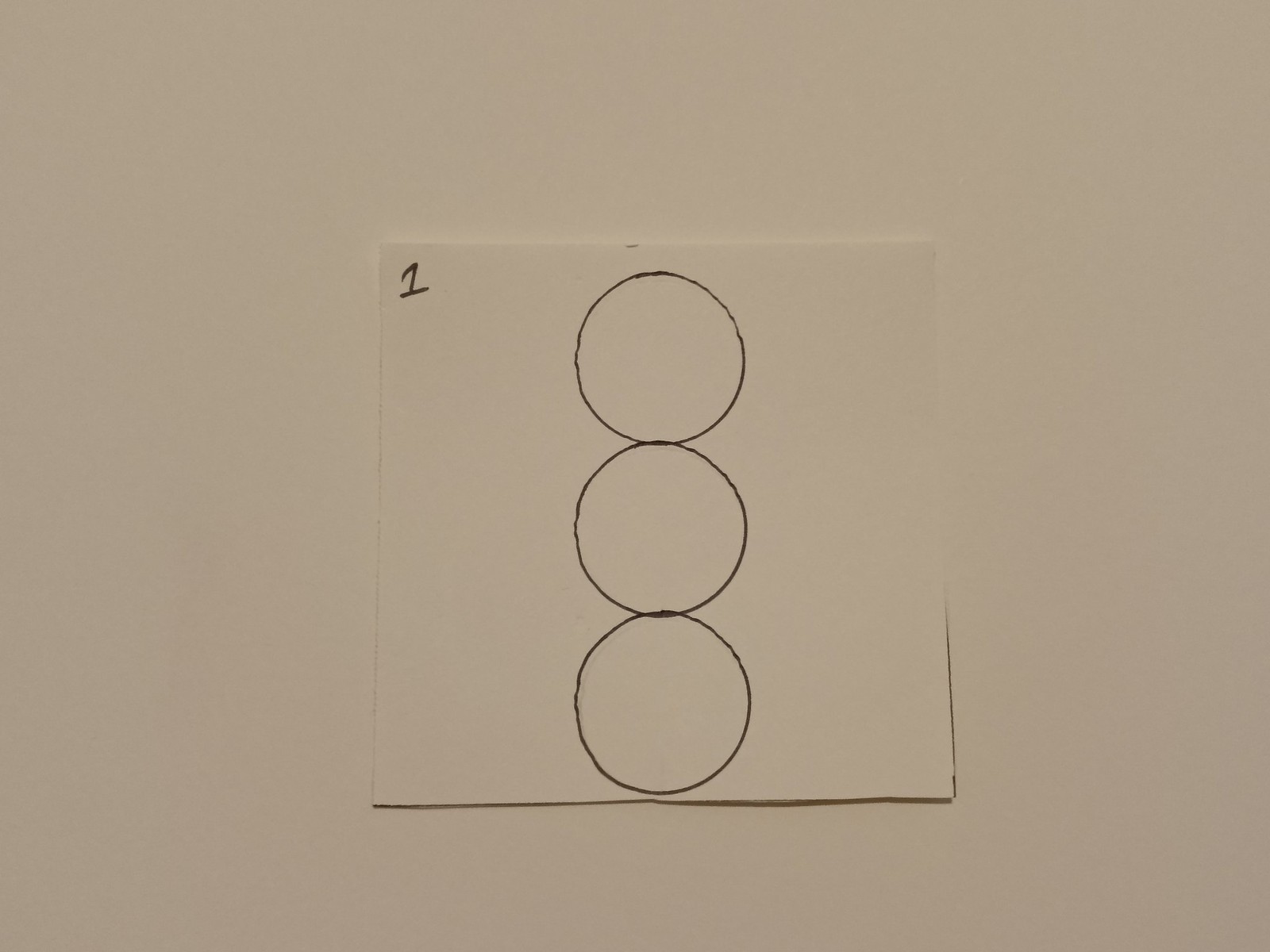The image displays a square sheet of paper resting on top of another piece of paper. The prominent boundary of the top square sheet is particularly noticeable along its lower edge due to a shadow effect, suggesting it isn't lying completely flat. A partial shadow is also visible along the lower half of the right-hand side. The remainder of the sheet's edges are less defined and require closer inspection to discern.

At the top center of the square sheet, there is a small mark of note. The sheet features three perfectly circular black dots, aligned vertically like traffic lights. These circles are contiguous, with no gaps or overlaps between them, each perfectly touching the next. The bottom circle is positioned almost at the edge of the sheet.

In the top left corner of the sheet, the number "1" is prominently written in black marker. There are no other markings or features on the sheet.